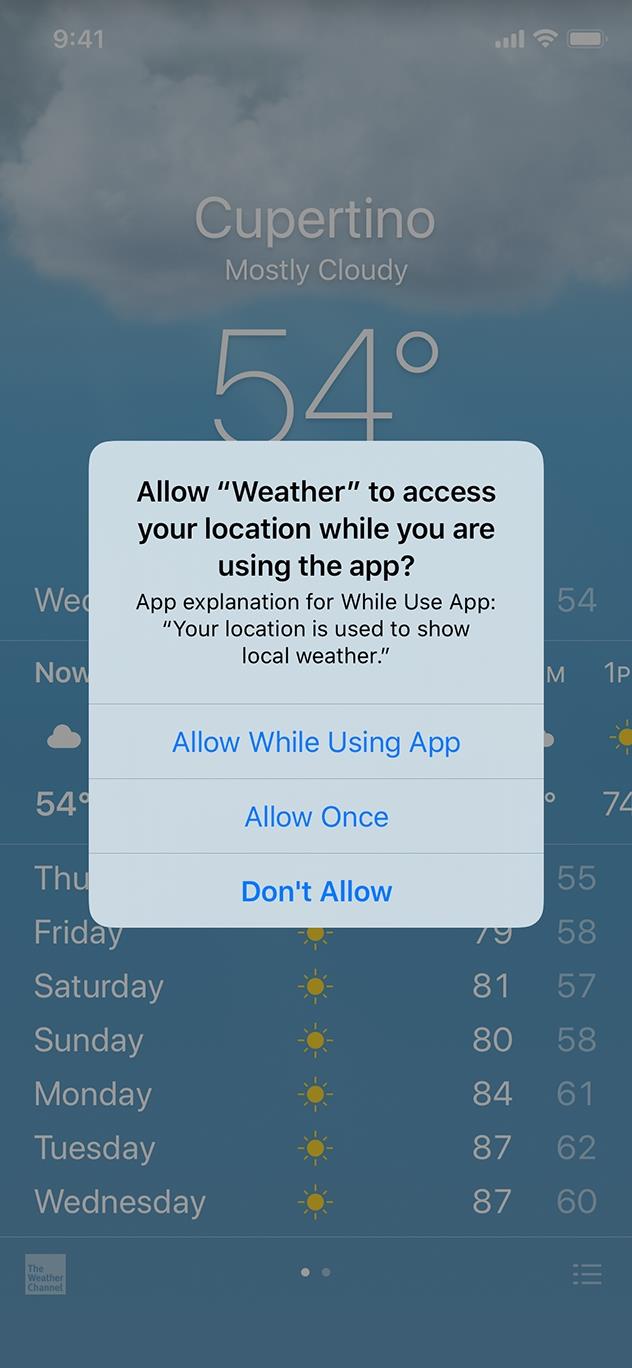**Detailed Caption:**

The image showcases a vertically oriented screenshot of a weather app taken from a smart device. The background features a serene gradient of sky blue transitioning from a lighter shade in the middle to a slightly darker shade towards the top and bottom, complementing the scattered white clouds.

In the upper left corner of the screenshot, the time is displayed as 9:41. To the right of this, the signal strength bars, Wi-Fi icon, and battery life icon are visible, providing a comprehensive view of the device's status.

The weather information for Cupertino is prominently displayed in large, clear white text. The app indicates that the current weather is "Mostly Cloudy," with a temperature of 54°F. 

Towards the top center of the screen, there's a dark translucent box asking for location access: "Allow Weather to access your location while you are using the app." Below this request, a less bold explanation states, "Your location is used to show local weather."

Three interactive options are listed in blue text within the box:
1. Allow While Using App
2. Allow Once
3. Don’t Allow (this option is slightly more bolded than the others).

Below this request box, the app continues to list the days of the week along with the corresponding temperatures for different times of the day, offering a detailed forecast for Cupertino.